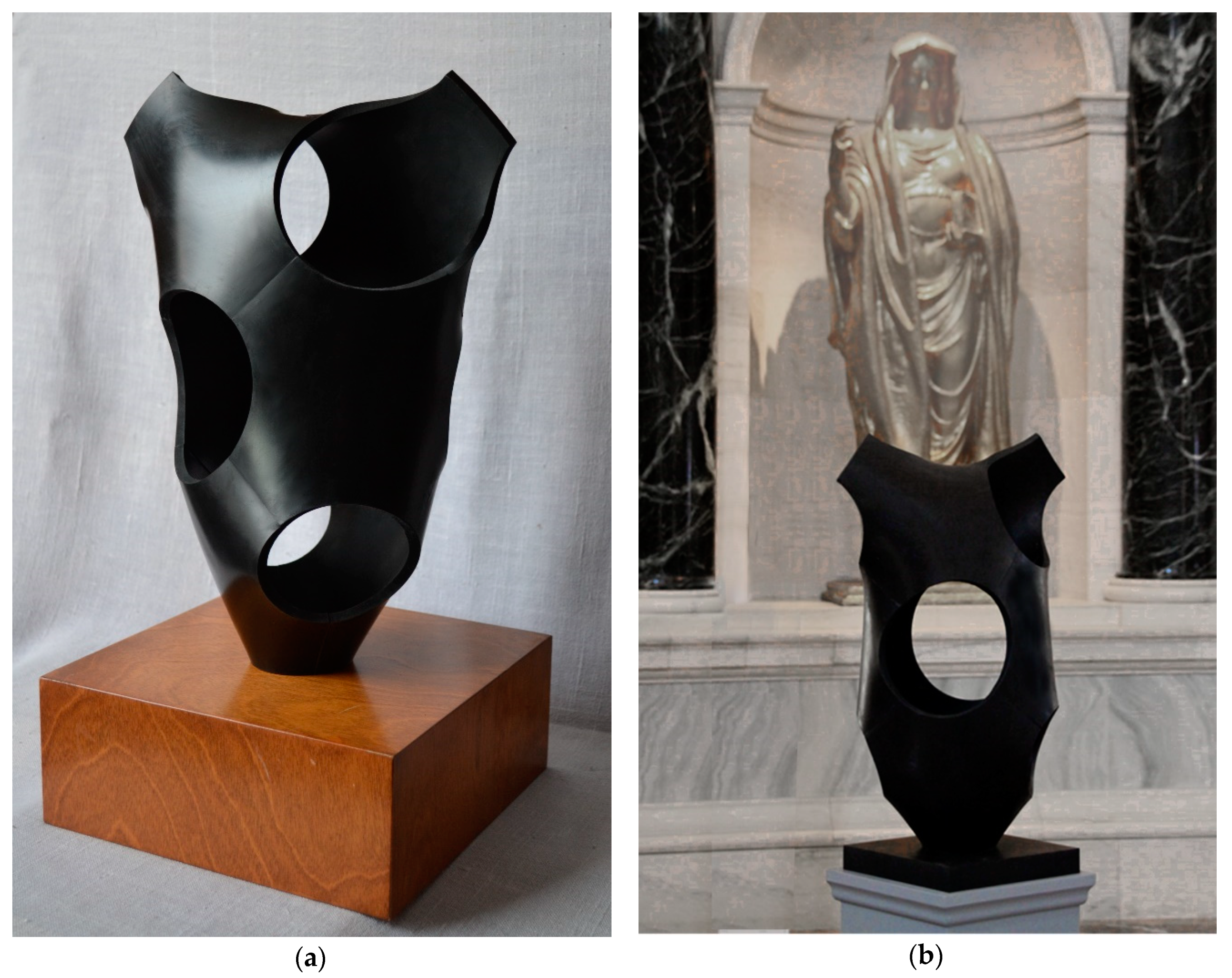Here is a refined and detailed caption for the photograph described:

---

**(A)** The left image features a modern black sculpture mounted on a polished wooden base. The wooden base, resembling half of a thick cube, is oriented with one of its corners facing the viewer. The medium-toned wood displays prominent grain patterns. The sculpture, which seems to be made of polished steel with a satiny black finish, mimics the shape of a human torso. It features shoulders or ear-like protrusions at the top, which are chopped off flat, creating a stark silhouette. The torso-like form includes several large cutouts: a prominent hole where the crotch of a leotard would be, a large oval opening under the left armpit extending toward the hip, and another substantial void in the top right area, possibly extending through to the back. The background consists of draped white cloth, enhancing the contrast and focus on the sculpture.

**(B)** The right image displays a similar modern sculpture, potentially the same piece viewed from a different angle or a different but closely resembling artwork. This sculpture stands on a sleeker white pedestal, set against an elaborate marble backdrop. The marble wall features various textures and colors, including an inset statue of the Madonna with an arm raised, dressed in flowing robes within an arch-shaped alcove. The juxtaposition of the modern black sculpture with the classical white marble statue and the richly grained marble wall creates a striking visual contrast.

---

This caption provides an organized and detailed description of each photograph and highlights the notable features and background elements.